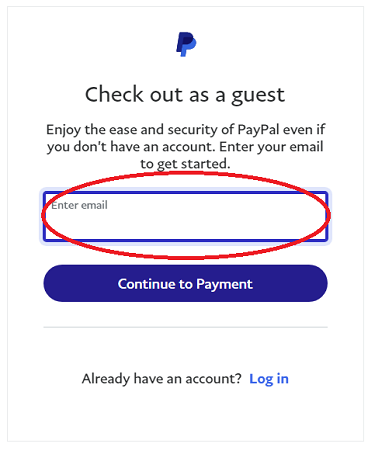In the upper section of the image, there is a prominent 3D letter "P" representing the PayPal logo. The logo features a darker "P" in the foreground and a lighter "P" in the background, creating a three-dimensional effect. Below the logo, in bold black text, the phrase "Check out as a guest" is displayed. Further down, another line of black text reads, "Enjoy the ease and security of PayPal, even if you don't have an account. Enter your email to get started."

A long blue rectangular input field is positioned beneath this text. Inside the rectangle, in small gray letters, it says "Enter email." The input field is circled in red, drawing significant attention to this area without the circle extending to the very edges of the rectangle.

Below the input field, there is a long blue button with white text that reads, "Continue to payment." Approximately three inches below this button, gray text asks, "Already have an account?" On the right side of this text, there is a blue "Log In" option with a capitalized "L."